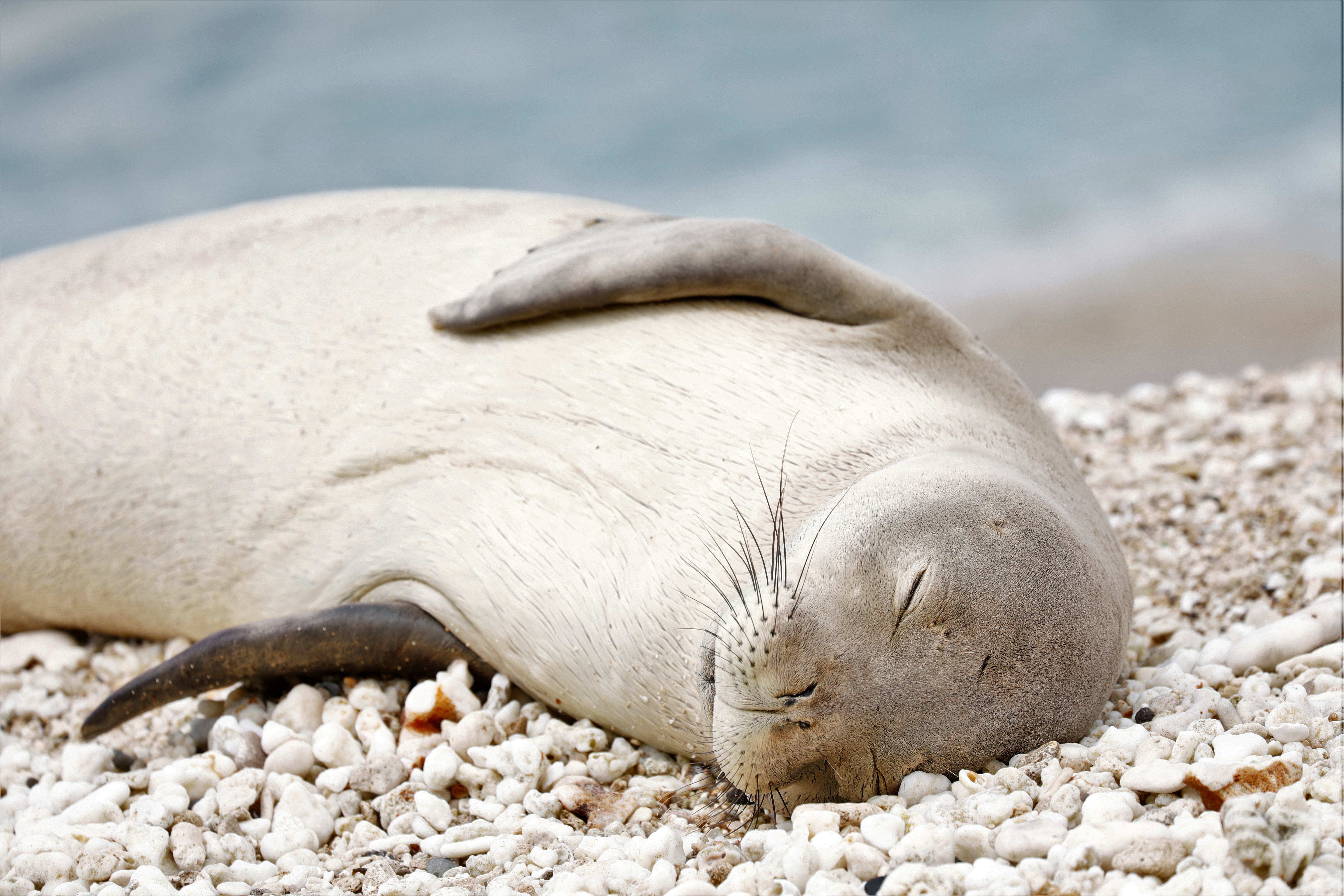This close-up photograph captures an adorable, young seal peacefully sleeping on white stones. The seal, primarily light gray with darker gray flippers and shadings of tan, has its head facing the camera, showcasing its meticulously detailed long whiskers and closed eyes. The subtle wrinkles on its off-white belly are visible as it rests on its side, with one flipper touching its belly and the other draped across the stones. There are noticeable scars on its head, including a long indentation on its forehead and a dent on the right side of its face. The background features a beautifully blurred outline of the ocean, with white caps crashing onto the sand, further emphasizing the tranquility of the scene.